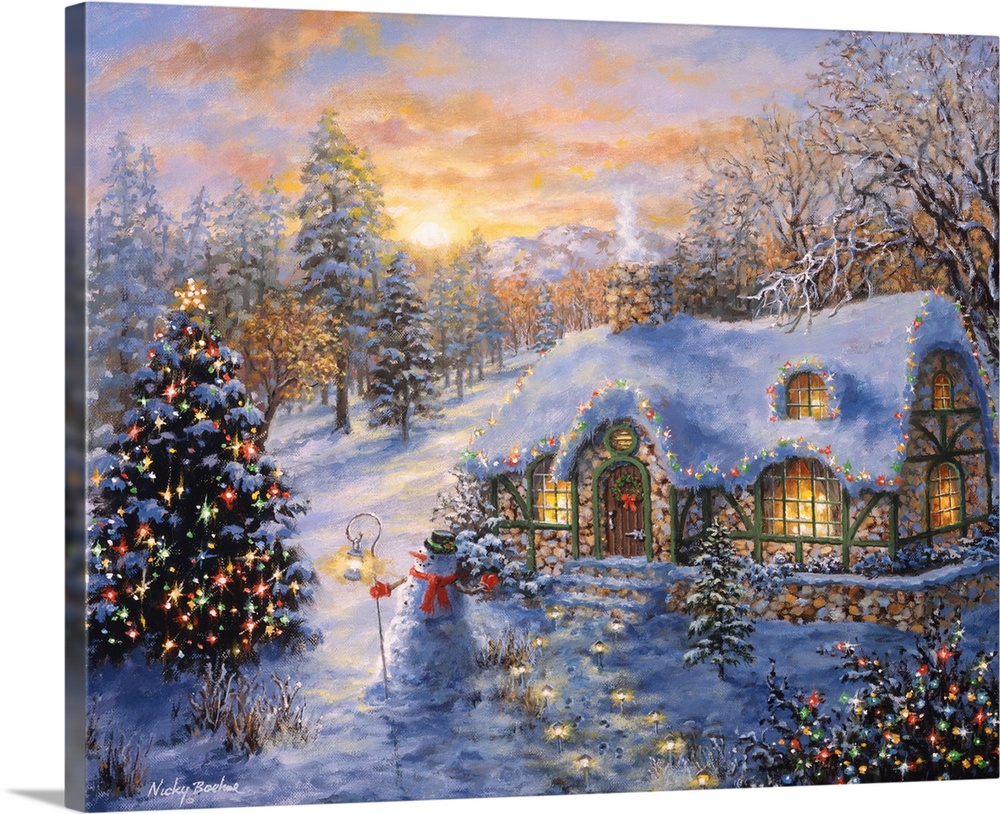This painting vividly captures a cozy winter scene, highlighting the festive spirit of Christmas. The central focus is a charming stone house, adorned with distinctive green outlines on its doors and windows, and a wooden brown door. Christmas decorations embellish its roof and the area in front of the door, complemented by a blanket of snow on the rooftop and a chimney releasing white smoke into the crisp blue sky. The sky itself is a picturesque blend of blue, orange, and yellow hues, suggesting a serene sunrise or sunset with a soft, light-yellow sun at its center.

In front of the house, a cheerful snowman stands out, donning a green hat, an orange scarf, and orange gloves. It holds a lamp in its right hand, adding a warm glow to the scene. To the right of the house, a Christmas tree sparkles with decorative lights and is crowned with a golden star, contributing to the festive ambiance. Snow-capped pine trees and distant white mountains add depth to the background, enhancing the wintry atmosphere.

Adding further detail, the bottom right corner of the painting includes shrubs illuminated with Christmas lights, while the bottom left corner features the artist's signature, Wookie, rendered in white. Overall, this painting encapsulates the peaceful yet joyous essence of a wintry Christmas scene.